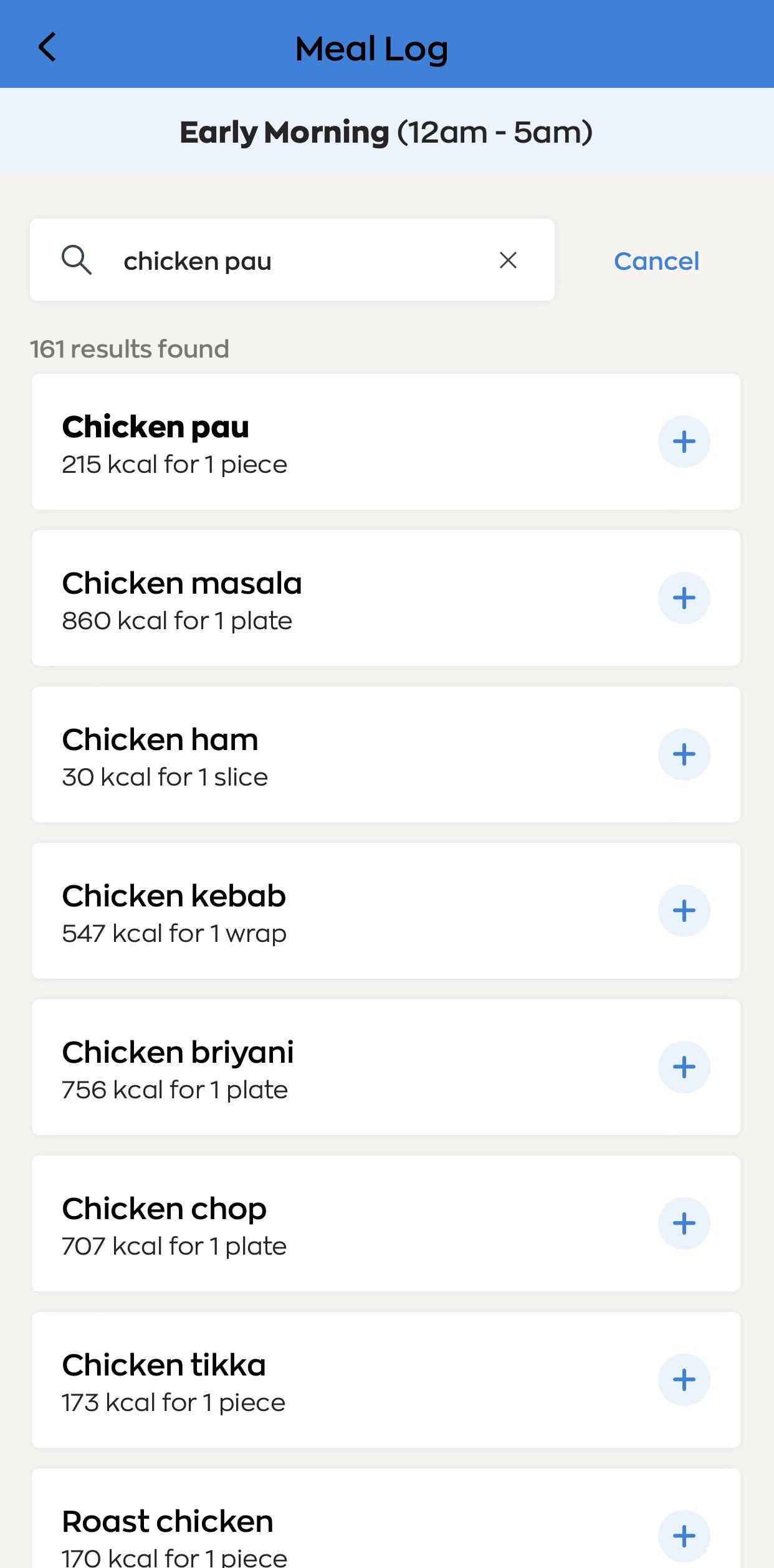The image is a vertically oriented rectangle with a blue banner at the top. Within the banner, "Meal Log" is written in black, accompanied by a left-pointing arrow. Beneath the blue banner, the background is light gray, displaying "Early Morning" in dark, bold black letters, followed by "(12am-5am)" in parentheses. Directly beneath, there is a search bar featuring a magnifying glass icon. Inside the search bar, the text "Chicken Pau" is written, with an 'X' at the right end for clearing the search. To the right of the search bar, the word "Cancel" is displayed in blue text. Below the search bar, an indication of "161 results found" is shown. The first result is "Chicken Pau," listed in bold, with a caloric information of "215 Kcal for one piece." Subsequent entries include "Chicken Masala," "Chicken Ham," "Chicken Kebab," "Chicken Biryani," "Chicken Chop," "Chicken Tikka," and "Roast Chicken," all listed below.